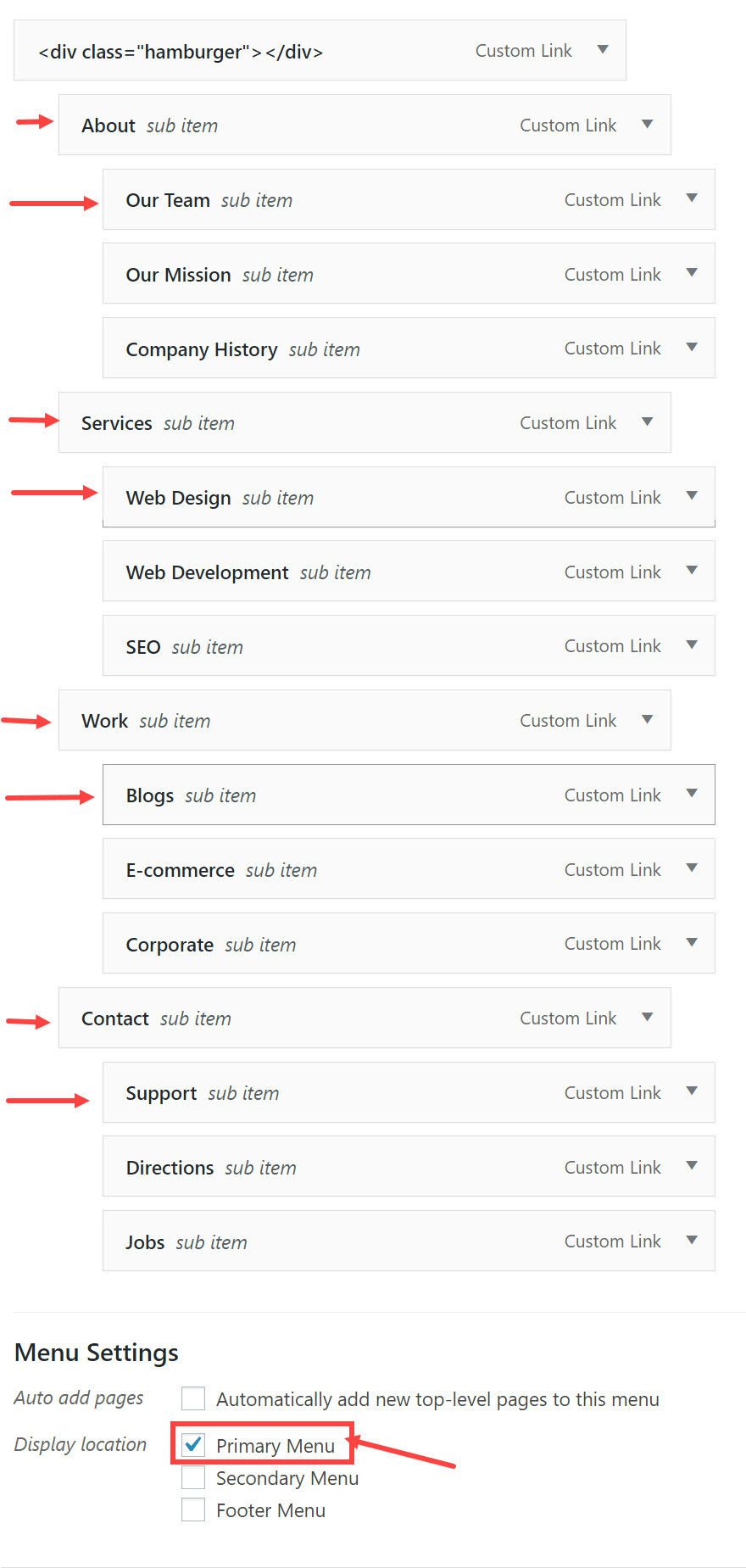This image is a screenshot from a webpage, specifically a utility page likely used for configuring a website menu. The background is predominantly white. The interface consists of a vertical array of very light gray, almost white, rectangles that function as drop-down menus. Each rectangle features the label "Custom Link" in light gray font, accompanied by an inverted gray triangle indicating the drop-down functionality.

On the left side of these rectangles, there are several menu items listed, starting from the top with "HTML," followed by "Hamburger," "About," "Our Team," "Our Mission," "Company History," "Services," "Web Design," "Web Development," "SEO Work," "Blogs," "E-commerce," "Corporate," "Contact," "Support," "Directions," and "Jobs." Some of these items have red arrows pointing towards them on the right side, possibly indicating they are selected or highlighted.

At the bottom of the image, in black text, there is a section labeled "Menu Settings." Below this, there is an option labeled "Auto Add Pages," with an instruction to automatically add new top-level pages to this menu. Further down, another section labeled "Display Location" includes a checkbox next to "Primary Menu," which is enclosed in a red rectangle and marked by an arrow pointing to it, signifying its significance or selection as the primary menu.